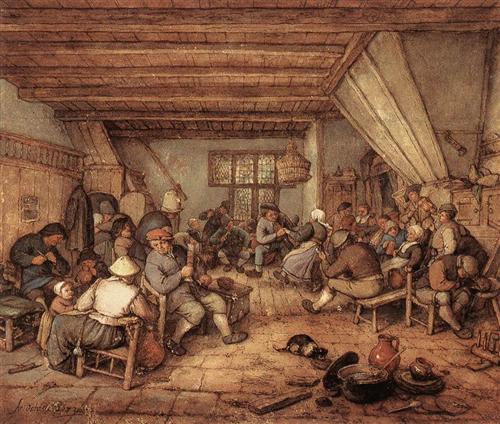The image depicts an old, medieval-style painting of a bustling, brown-toned interior scene. The room, characterized by its wooden ceiling with exposed beams and sections of stone and ceramic-tiled flooring, is filled with commoners of all kinds—men, women, and children. People are gathered around the edges of the room, sitting on wooden chairs and engaging with one another. In the center of the space, there is a cat drinking from a bowl on the floor, surrounded by pots and pans. Toward the back right, a hanging birdcage can be seen above a man in a blue hat, situated near a small window. The right wall features a fireplace, and a lantern hangs from the rafters above. On the left side, a front door is visible as people dance and socialize, creating a lively, tavern-like atmosphere.